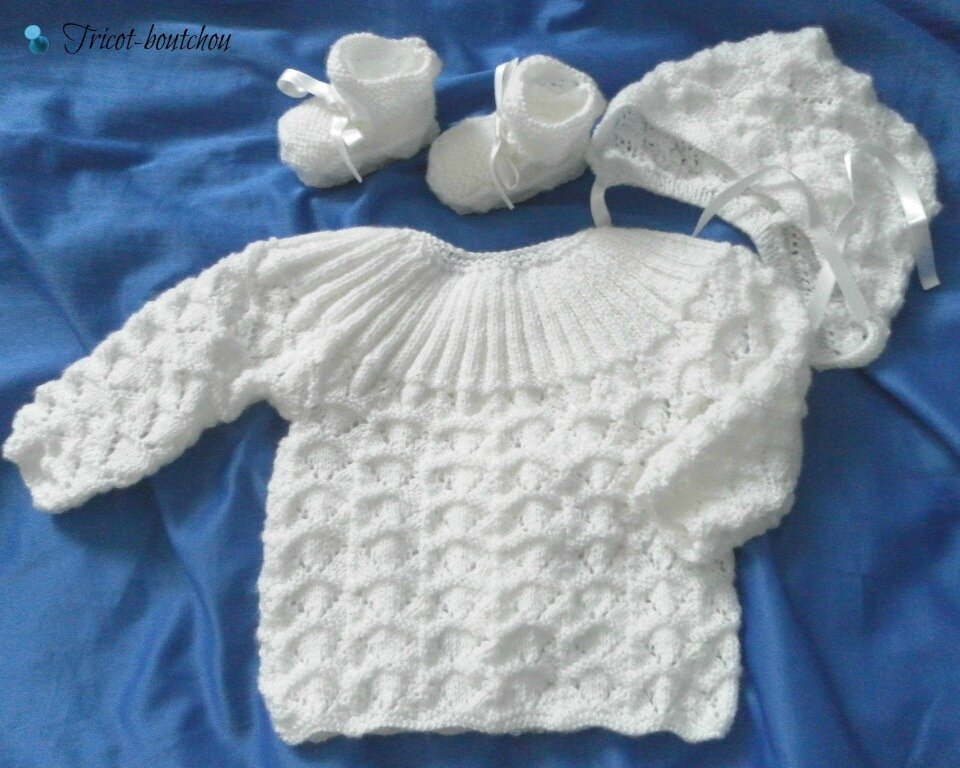This top-down image showcases a beautifully hand-crocheted newborn outfit, set against a rippled medium blue bed sheet background that adds texture and depth. The centerpiece is a decorative white sweater, intricately designed with a patterned collar around the shoulders and neckline, occupying the middle and bottom two-thirds of the frame. Above the sweater, arranged thoughtfully, are matching accessories: two small booties to the left, both adorned with white bows and positioned at a slight angle, and a bonnet in the upper right corner, complete with white tie strings for securing around the baby’s head. To the top left of this carefully assembled display, the watermark 'Tricot Bouchot' is visible, accompanied by a blue thumbtack. This lovingly crafted, homemade set evokes a sense of warmth and coziness, perfect for a newborn.